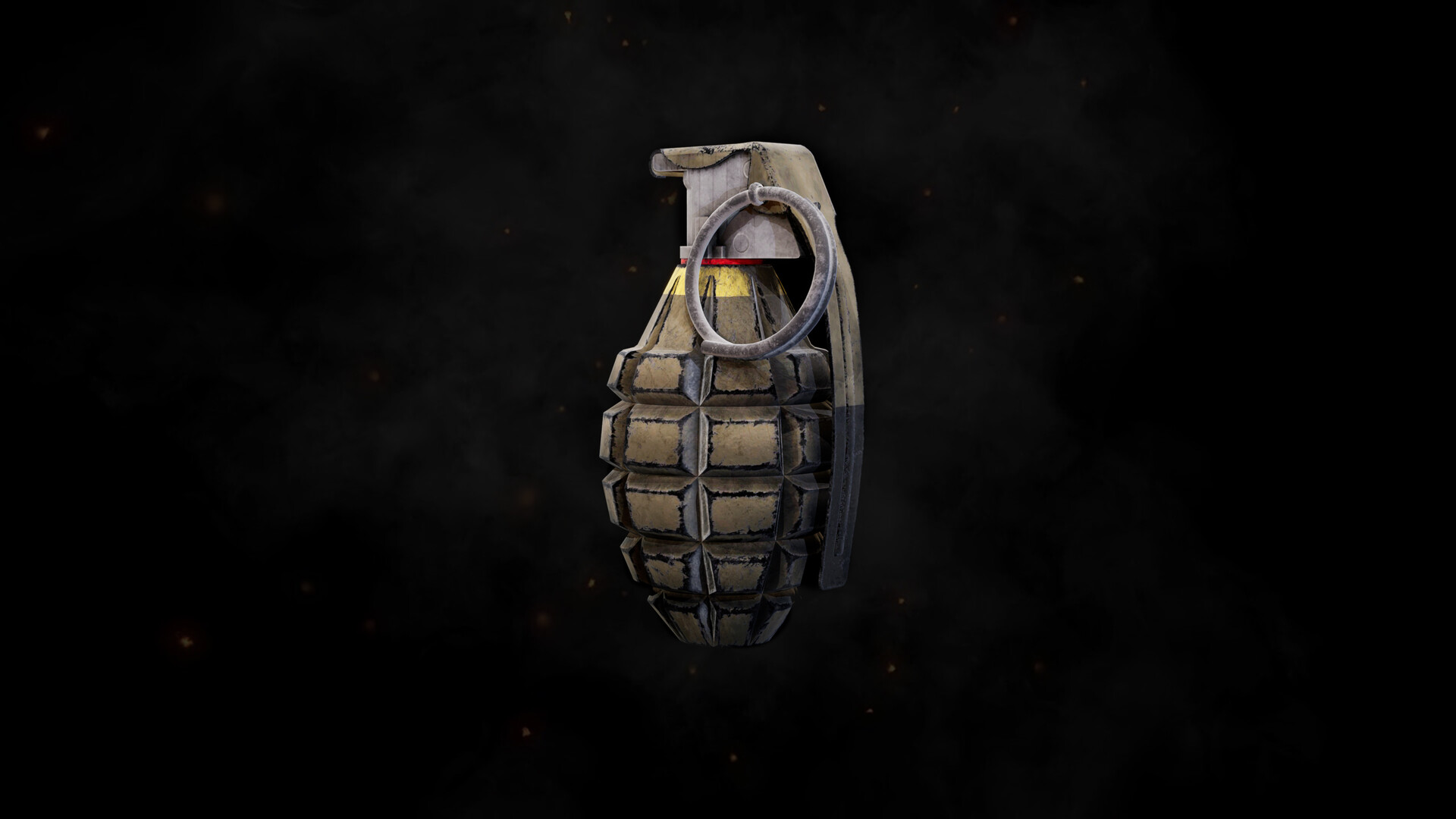The image features a digital illustration of a grenade positioned centrally against a completely black background. The grenade, displaying a standard egg-like or lemon shape, is fully visible and notably textured with worn detailing. Its greenish body is characterized by rectangular spokes and vertical columns of five protruding bumps each, giving it an aged and rugged appearance. The metallic grip of the grenade shows signs of rust, with black spots scattered across its surface. The grenade's silver ring, part of the pin mechanism, appears equally worn, suggesting it has not been recently pulled. A subtle red band encircles the grenade just below the metal top, which is predominantly steel gray and merges into a lower black handle. A faint smoky outline surrounds the grenade, possibly adding to its vintage or advertisement-like aura. This meticulously crafted illustration emphasizes the grenade's realism and aged condition, highlighting both its utilitarian design and evocative visual appeal.